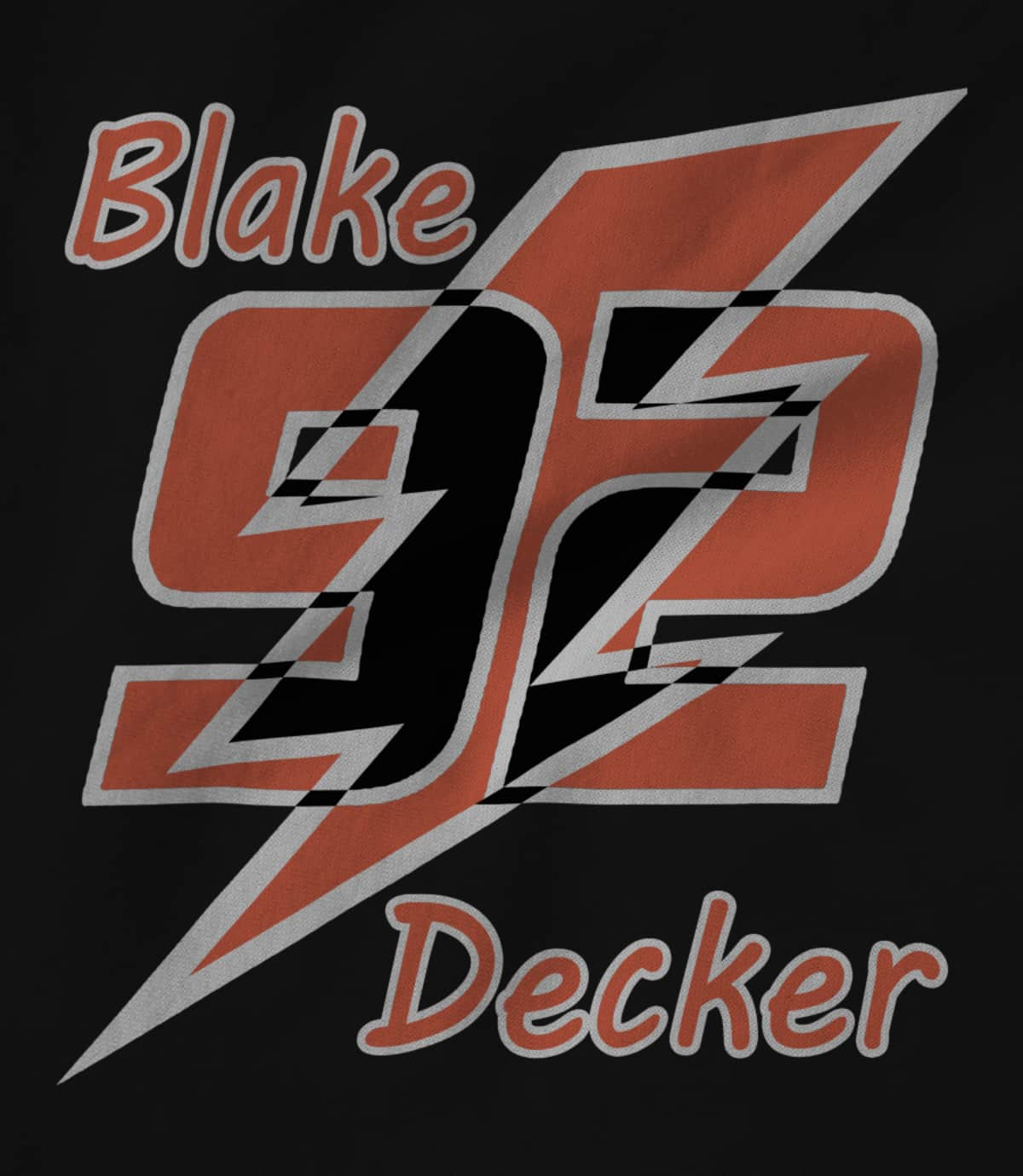The image features a black background with the name "Blake Decker" and the number "92" prominently displayed. In the upper left corner, the word "Blake" is written in a red font with a gray outline, and in the lower right corner, the word "Decker" appears in the same style. The center of the image is dominated by the number "92," which is also in red with a gray outline. A prominent lightning bolt cuts through the number "92," turning the intersected areas of the numbers black. The background of the lightning bolt itself is bright red, adding a striking contrast. The overall color scheme features a dominant black, accented by shades of red that have a faded, orange-ish tint, and light gray outlines. The vivid imagery and dynamic design suggest a racing or sports theme, possibly alluding to a race car driver's number and name.